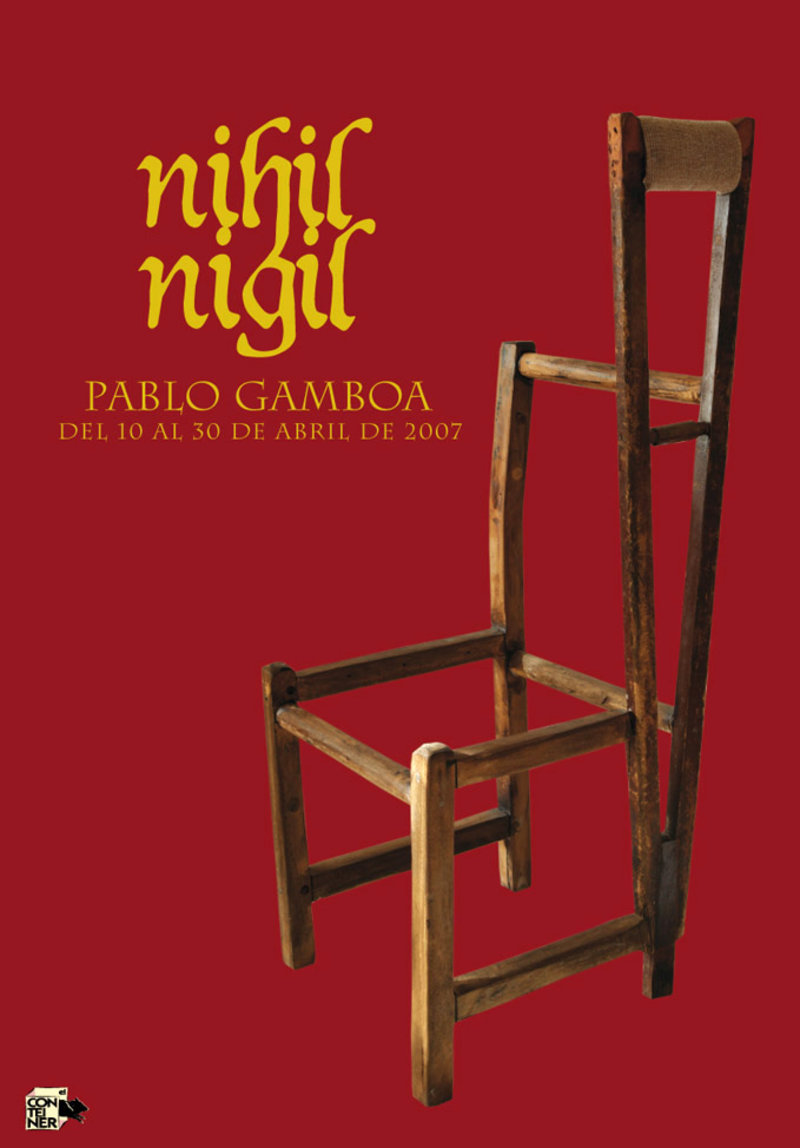The image appears to be an advertisement or book cover with a red background and yellow text. The text at the top reads "Nihil Niggle" followed by "Pablo Gamboa," and beneath that, it says "Del 10 Al 30 De Abril De 2007," indicating an event that took place from April 10 to April 30, 2007. The prominent feature of the image is a distinctive wooden chair. The chair is high-backed and partially deconstructed, with a notable wooden crutch integrated into the left side, serving as both a leg and part of the backrest. The unconventional design of the chair captures attention due to the stark contrast between the traditional wooden elements and the oddly placed crutch, which replaces the standard structure on one side, making the chair appear both familiar and unusual.